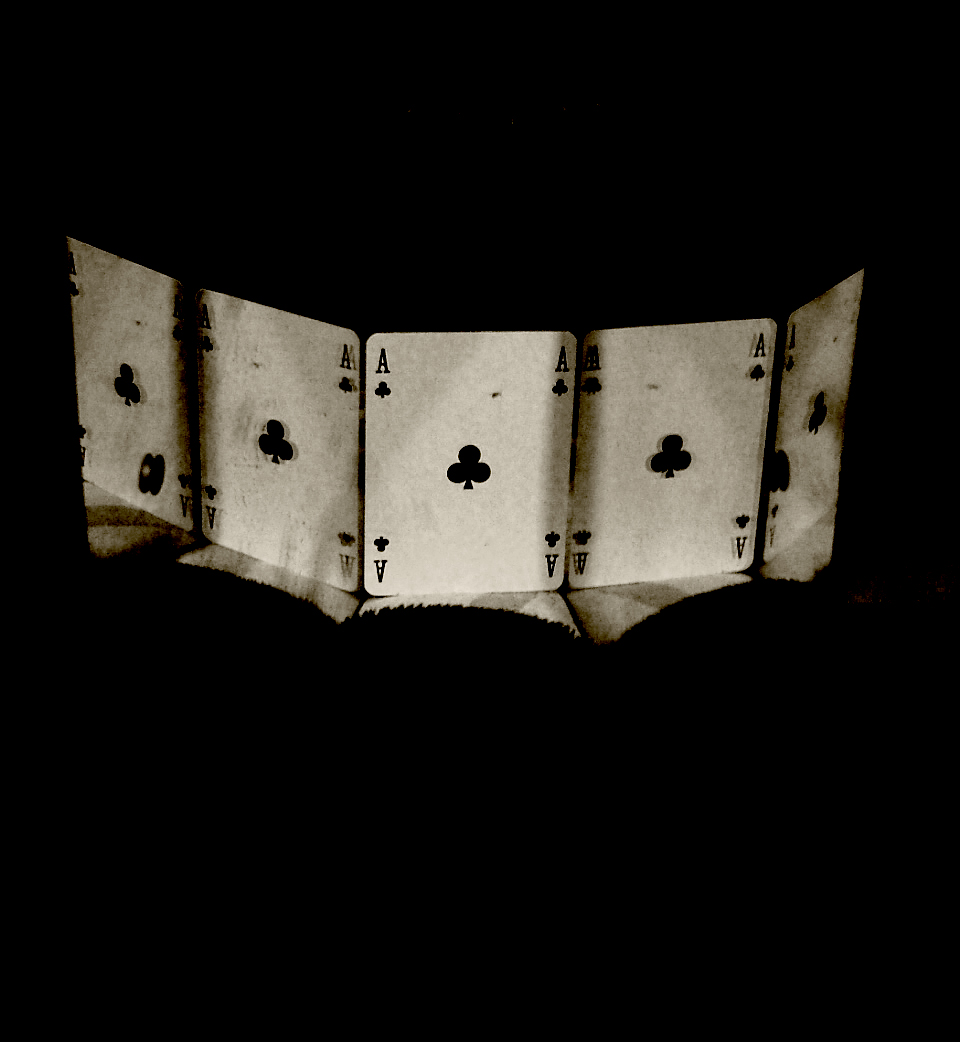The image presents an intriguing composition that blurs the line between reality and digital art. Five identical Ace of Clubs playing cards stand vertically in a closely arranged formation, slightly skewed to form a subtle arc that resembles a delicate wall. The cards are backlit, casting a faint reflection beneath them, adding to the surreal quality of the scene. The exposure is intentionally off, lending a dreamlike, almost eerie atmosphere to the image, with the background fading into deep black, isolating the cards from any discernible context. The focus is soft, further enhancing the mysterious aura. Each card features the classic design: a central club symbol surrounded by the letter 'A' and smaller club icons in the corners. The pattern beneath the cards is mirrored and abstract, perhaps a reflection or an artistic element, contributing to the image's enigmatic and avant-garde feel.